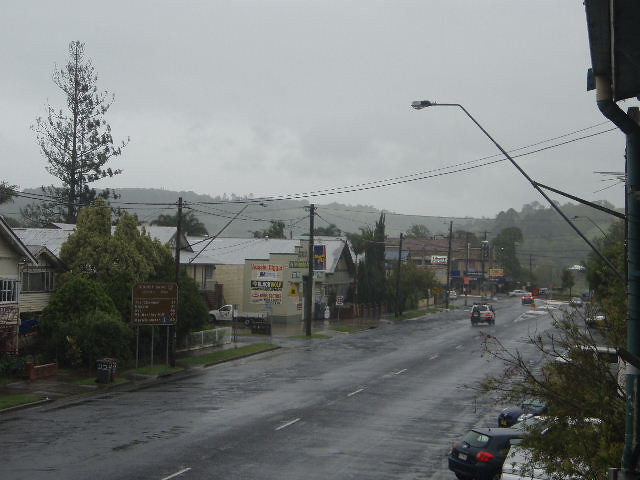This color photograph captures a rainy day on what appears to be the main street of a small town, oriented in landscape format. The dark, cloudy sky and wet pavement indicate it has recently rained. The street, which widens in the foreground and narrows towards the horizon, is lined with parked cars on the right-hand side. Several buildings and small businesses, including what looks like a hotel, are visible on the left side of the road, interspersed with tall trees and streetlamps, and connected by telephone wires. In the background, a mountain range looms, shrouded in gray mist. To the right in the foreground, there is a large tree branch, partially obscuring a few parked vehicles, and a streetlamp on a dark metal pole. An intersection is visible at the end of the street, where additional buildings and possibly a sizable metal silo stand. Everything is rendered in detailed photographic realism, capturing the quiet, drizzly atmosphere of the town.